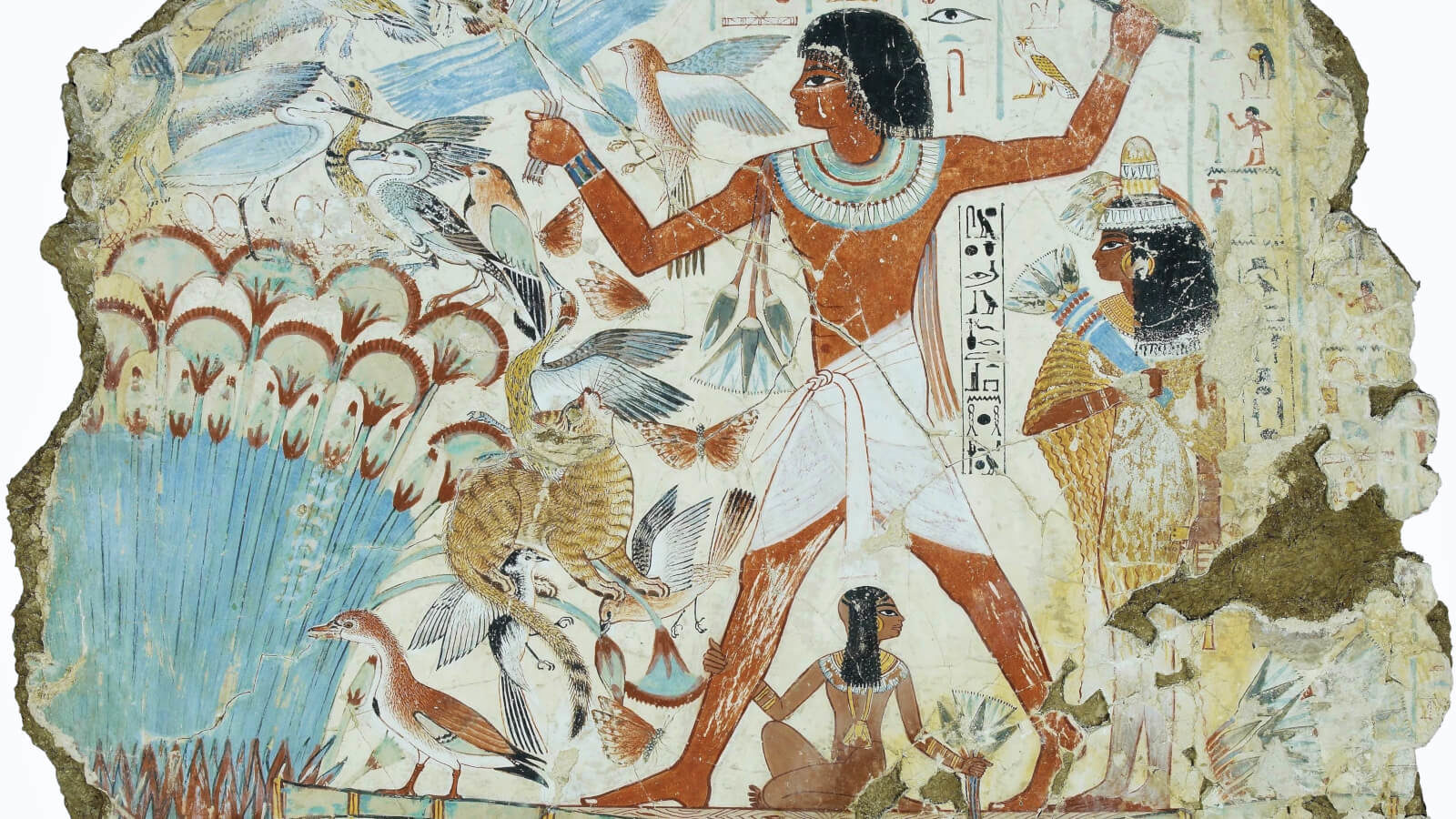The image is a horizontal rectangular plaque or stone with a vivid painting in Egyptian style, bordered by irregular broken edges on both sides and straight borders on the top and bottom. Dominating the right side of the frame is a male figure with brown skin, wearing a loin cloth and a white necklace. It's unclear whether the figure dons a helmet or has hair. The man is depicted mid-step, and beneath his stride, there is a smaller seated woman with her back turned to the viewer. To his right is another partial figure, and to the left, the image includes additional elements such as reeds and a stream running across the top section. The middle section features various hieroglyphics and ornamental symbols in black. Animals such as an ibis, ornamental birds, and a cat are prominently displayed throughout, suggesting a rich natural scene or possibly a map. A minor character, a child, is depicted clinging to the man's leg. The depiction is ornate and clear, enriched by natural light that highlights the vivid colors and details of the scene.